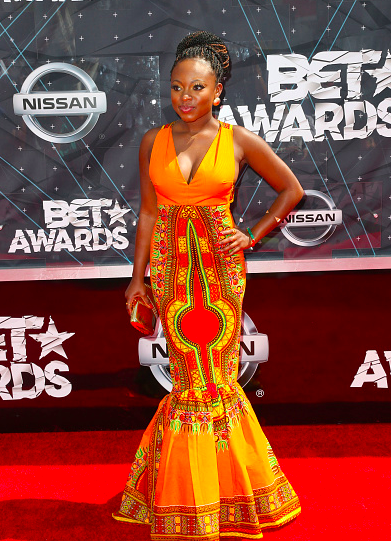In this vibrant red carpet photo taken at the BET Awards, the scene is set with a backdrop showcasing the logos of BET Awards, complete with a star, alongside Nissan, against a primarily white and gray background, accented with a striking dark red layer at the bottom. The floor features a bright red carpet that adds to the glamour of the event. Captured at the center, the woman is African American and exudes elegance in a mermaid-style dress. The top of her dress is a bold orange, while the lower part showcases intricate floral patterns in red, yellow, purple, and green. She accessorizes with large red and white circular earrings, and a green bracelet on her wrist, which is stylishly placed on her hip. Her hair is neatly pulled back into a bun with a hint of orange braided in, and she carries a petite, presumably gold, clutch in her other hand. She gazes slightly off to the side, her smile illuminated by the camera flashes, embodying poise and sophistication against the event’s luxurious backdrop.